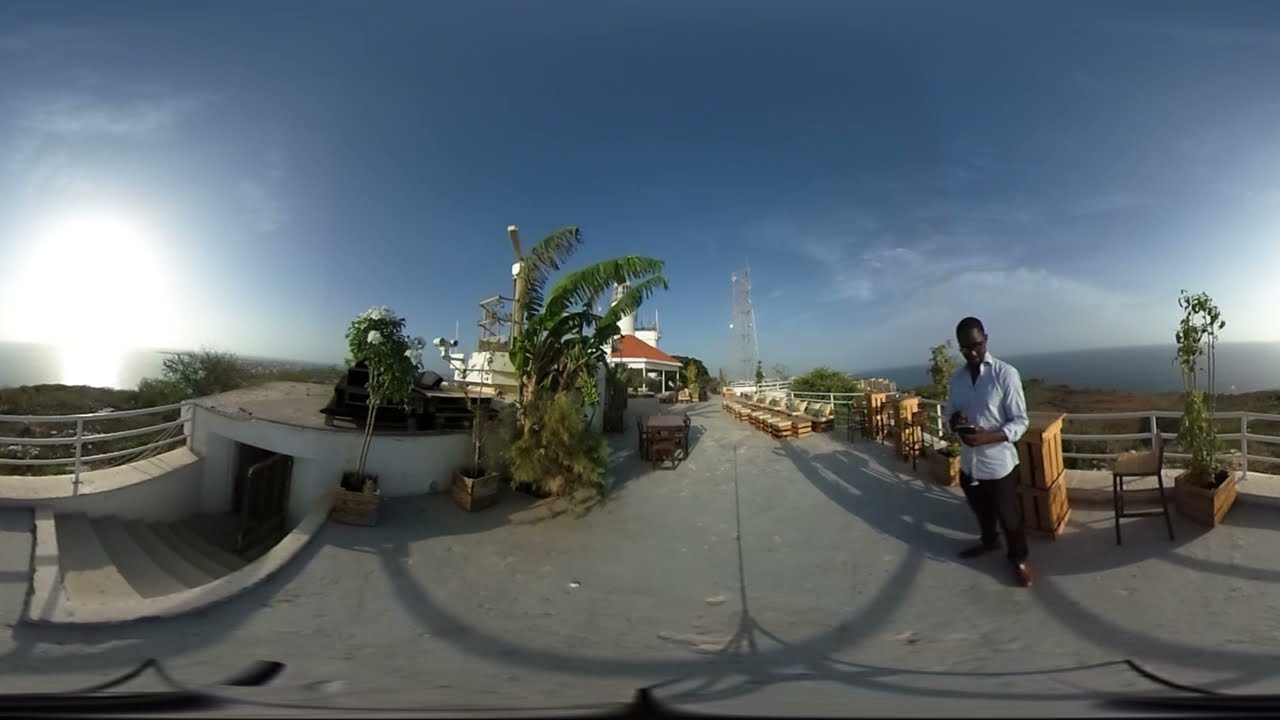This outdoor photograph, captured with a fisheye lens, provides a panoramic view of an elevated concrete walkway under a blue sky with scattered clouds. At the center right stands a young man of African descent, wearing a long-sleeved, untucked white shirt and black slacks. The curvature at the bottom of the image hints at the wide-angle effect of the lens.

The expansive scene depicts key elements on both sides. On the left, there is a bright sun appearing twice due to the panoramic effect, accompanied by a distant, grassy coastline leading out to the ocean. Below, a staircase leads down into a white building, and potted palm trees are situated along the walkway. Further along, there seems to be a small chapel or structure nestled behind the trees.

To the right, another stretch of the coastline and ocean is visible. In the distance, several structures can be seen, including what appears to be a communications or radio tower. Scattered chairs occupy the scene, emphasizing the area's open and communal nature. The image suggests it was taken during the late afternoon, given the low position of the sun in the sky.